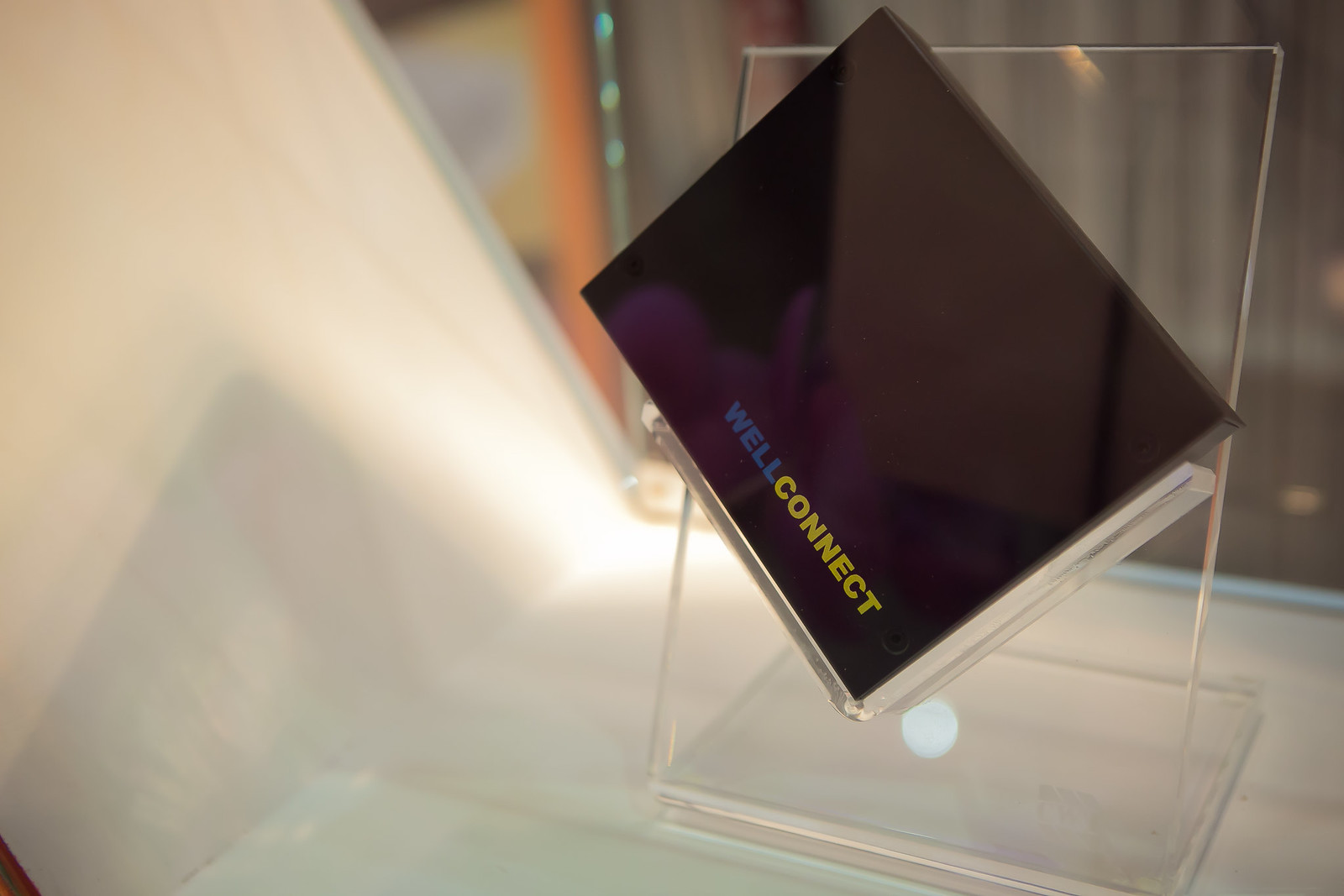The image depicts a display set atop a white countertop, with a somewhat confusing and hazy background on the left side. The background appears to show an orange vertical wall with some yellow to its left. Centrally positioned on the right side of the photo is a transparent plexiglass stand, angled back, upon which rests a black square object, possibly a box or book, with gray and purple accents. This object is oriented diagonally from the top center-left to the right. The lower right corner of the black object prominently features the words "well" in blue and "connect" in yellow. The display, likely related to computer technology or connectivity, appears clear and is sharply contrasted against the white countertop and the hazed backdrop.